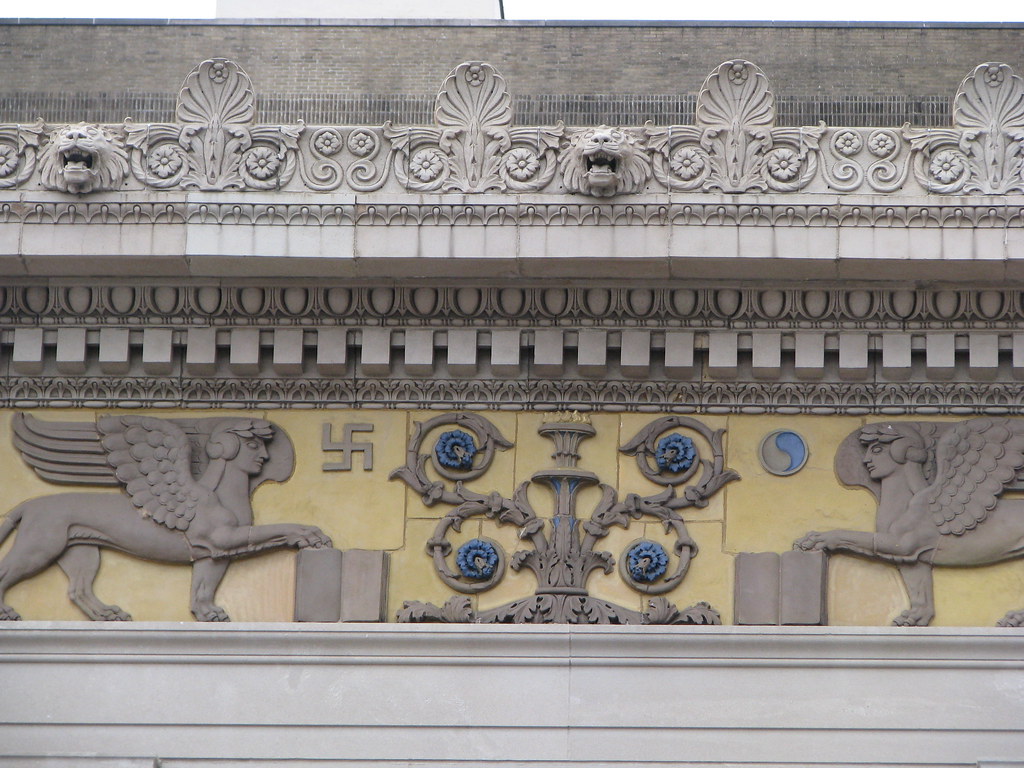The image displays a detailed section of a building's facade, showcasing a blend of architectural and decorative elements. The structure, presumably made of cement and adorned with white marble accents, features a beige or yellowish background. Intricate carvings and engravings embellish the upper portion, including a series of lion heads with open mouths. Below the marble ledge, a fascinating array of symbols and mythical figures are depicted.

Central to the composition is a sculpture resembling a torch or a fountain, with spiraling floral decorations transitioning from brown to blue. Flanking this centerpiece are two mythical creatures; each possesses the body of a lion, the wings of an eagle, and a human head, and their paws rest on open books. These figures, often described as griffins or pegasi with human heads, mirror each other on either side of the fountain.

To the left of the central sculpture, a swastika is engraved, seemingly the ancient, pre-20th-century version that is less controversial. On the right, a yin-yang symbol is present, with a blue right side and a brown left side.

The overall composition is rich in its Victorian-inspired patterns, combining various cultural symbols and motifs. The detailed artistry and the intricate mix of symbols suggest a significant cultural or religious context, potentially related to Buddhist or Hindu influences. The cement facade, devoid of ink or paint, relies on its engraved details to create a visually compelling and historically resonant design.